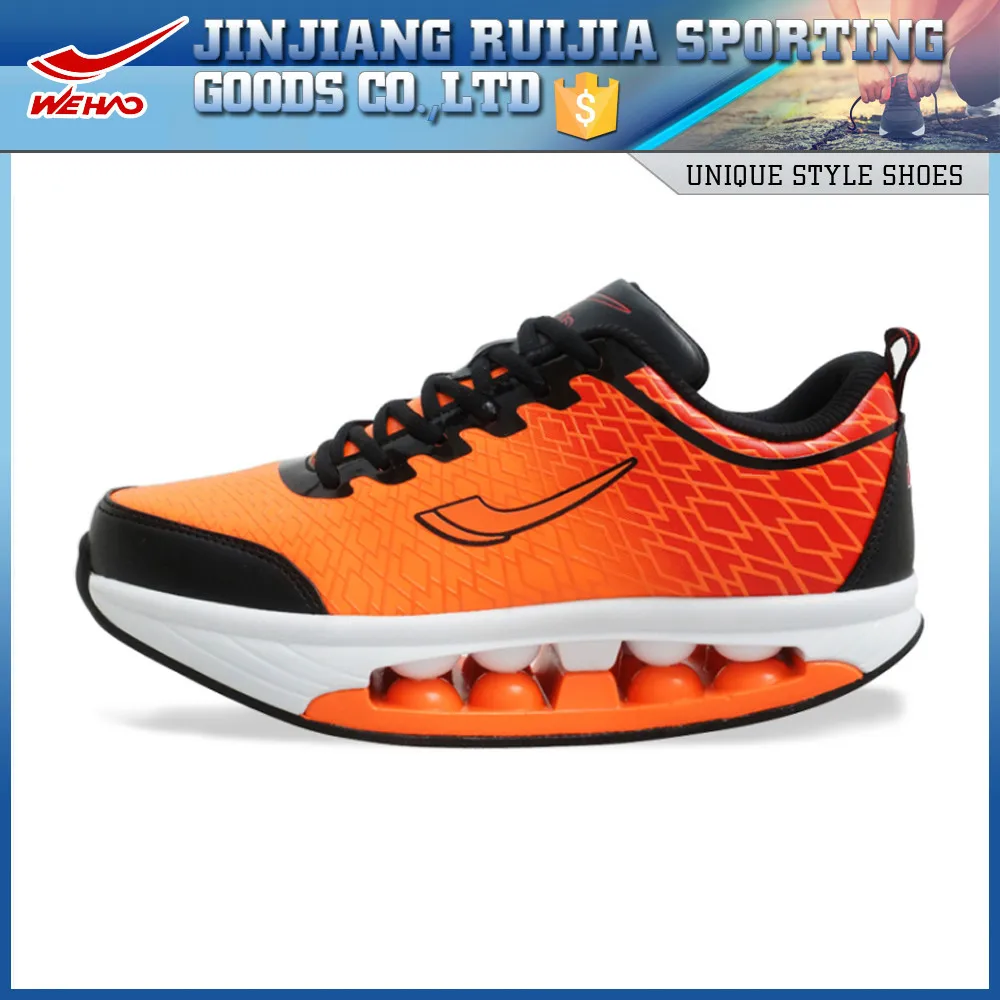This advertisement, surrounded by a gradient blue border transitioning from light at the top to dark at the bottom, showcases a unique athletic shoe. A prominent banner runs across the top, featuring a red checkmark on the left followed by "W.E.H.A." Next to this, in the center, the company's name is spelled out: "Xinjiang Rouge Sporting Goods Co., Ltd." To the right, there's a yellow badge with a white dollar sign, coupled with an image of a person, visible from the knee down, tying their shoe.

Below the banner, "Unique Style Shoes" is inscribed in small black lettering on a gray background. The main section of the image is dominated by an orange and black sneaker. This shoe features a strikingly curved sole designed for a rocking, cushioned gait. The sneaker showcases an orange body with black accents on the laces, tongue, and back, alongside white and orange highlights on the sole, providing not only distinctive style but also enhanced comfort and ergonomic design.